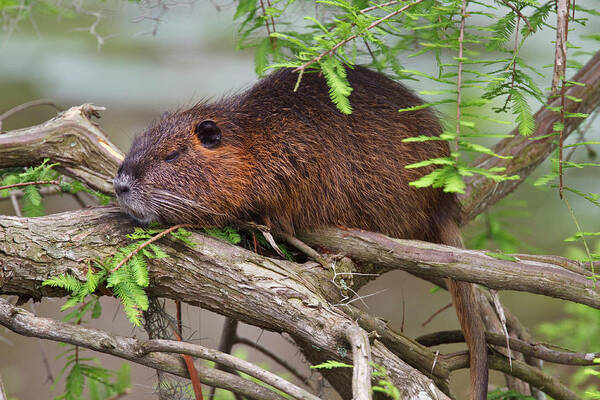In this detailed photograph, a brown-furred muskrat is resting on interwoven mangrove roots, blending seamlessly into its natural environment. The image, taken in an outdoor setting, showcases the muskrat's distinctive features: its smooth, thick, bare tail, white whiskers, and small, circular darker brown ears. Its eyes appear to be partially closed, adding to a tranquil or resting demeanor. Overhead, delicate green foliage hangs down, enhancing the natural ambiance with a blurred watery backdrop in the distance. The side profile of the muskrat reveals its rodent-like characteristics, including a beady black eye and a fur coat that subtly mixes brown and reddish hues, allowing it to camouflage effortlessly amongst the light brown branches.